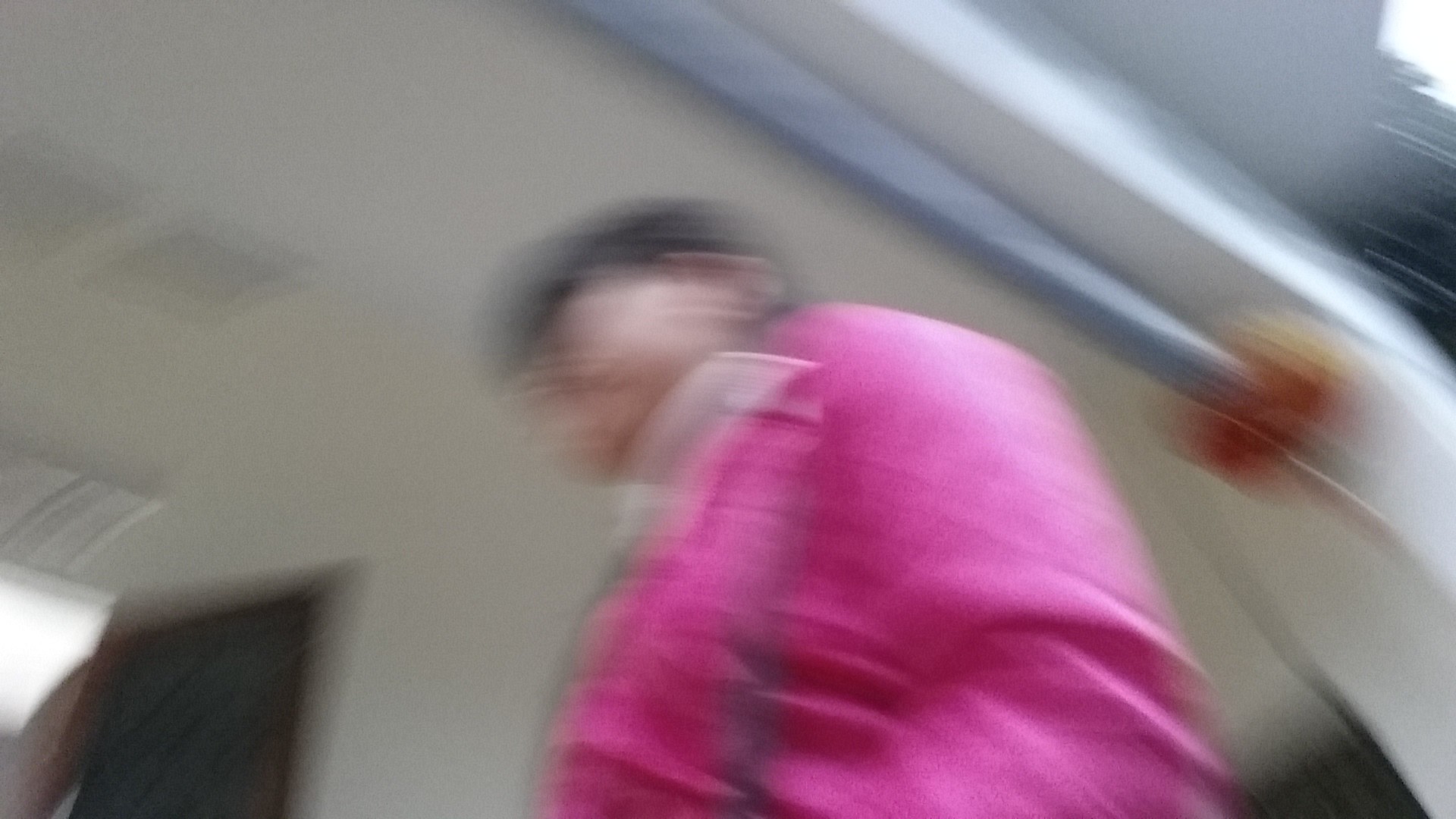In this very blurry image, the focal point appears to be a man in motion. He is wearing a traditional-style cap with a brim, reminiscent of the ones often worn by older gentlemen, possibly one from England. His outer garment, which could be either a shirt or a jacket, is a vivid hot pink, though the motion makes it difficult to distinguish. Above the garment, a white object is visible, but it's unclear if it is part of his attire or something he is carrying. The man has fair skin and short gray hair, though his face is indistinct due to the blur from the movement. There is a lighter patch around his chin that might be a beard. 

Overhead, there is a metal rod with a red object at one end, set against a white ceiling. The ceiling also features several grills. In the top left corner, a black object appears to be hanging down from a doorway. Additionally, a light source is visible in the image. Despite the indistinct details, the man and his rapid movement remain the central elements of the photograph.